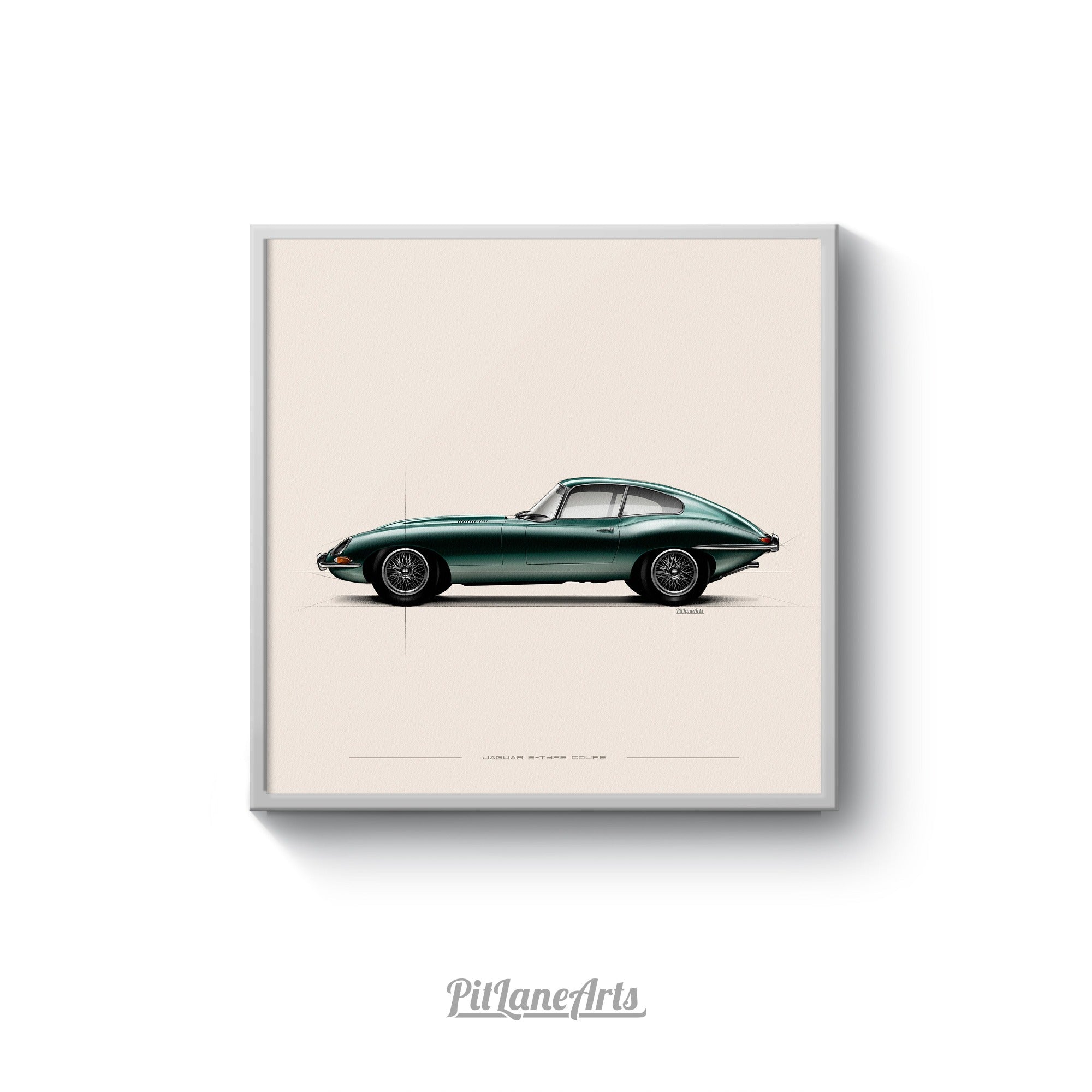This is an image of a sleek, aqua green sports car, possibly an older Corvette, facing left. The car features a darker green color down the middle, lighter green on the roof and below the doors, with spoked chrome wheels. The background of the image is completely white, casting a faint shadow beneath the car. The artwork, set within a red frame, features a white border and a tan interior. At the bottom of the image, there is some illegible black text and a small sign that reads "Pit Lane Arts" in cursive gray, suggesting the creator or vendor of the artwork.